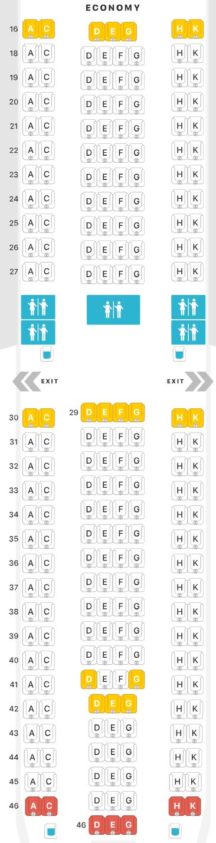The image depicts a website featuring a layout of multiple tables organized in a structured manner. It appears to showcase screenshots of two different pages, each divided into three columns. 

The first screenshot prominently displays the title "Economy" at the top. The small print makes the numerical details difficult to discern. Each column has a pair of golden-colored blocks at the top. The first column is labeled "AC," with repeated "AC" blocks beneath it—specifically, ten white "AC" blocks followed by two small blue boxes containing white penguin icons at the bottom of each row. Adjacent to this, there are numbers that are unreadable. 

In the middle section of the screenshot, the header appears to show the letters "D, E, G" at the top. Below this header, there are four columns labeled "D, E, F, G," each containing ten white blocks with corresponding letters and two blue boxes with white penguin icons at the bottom of each column. The last column is titled "H, K" in gold, and beneath it are ten white boxes labeled "H, K," with each row also ending in two small blue boxes with white penguin icons.

The second screenshot follows a similar pattern. The top is marked with golden blocks labeled "AC," and the columns beneath it are filled with white blocks labeled "AC," ending in red boxes at the bottom of each column. The middle columns are labeled "D, E, F, G," but halfway down, it switches to just "D, E, G," with red boxes at the bottom as well. The final column mirrors the previous with "H, K" at the top in gold, and white blocks labeled "H, K" descending with red boxes at the bottom.

In summary, the website showcases detailed tables with repeating patterns of labeled blocks and color-coded sections, although the exact numerical data is not clearly visible in the image.